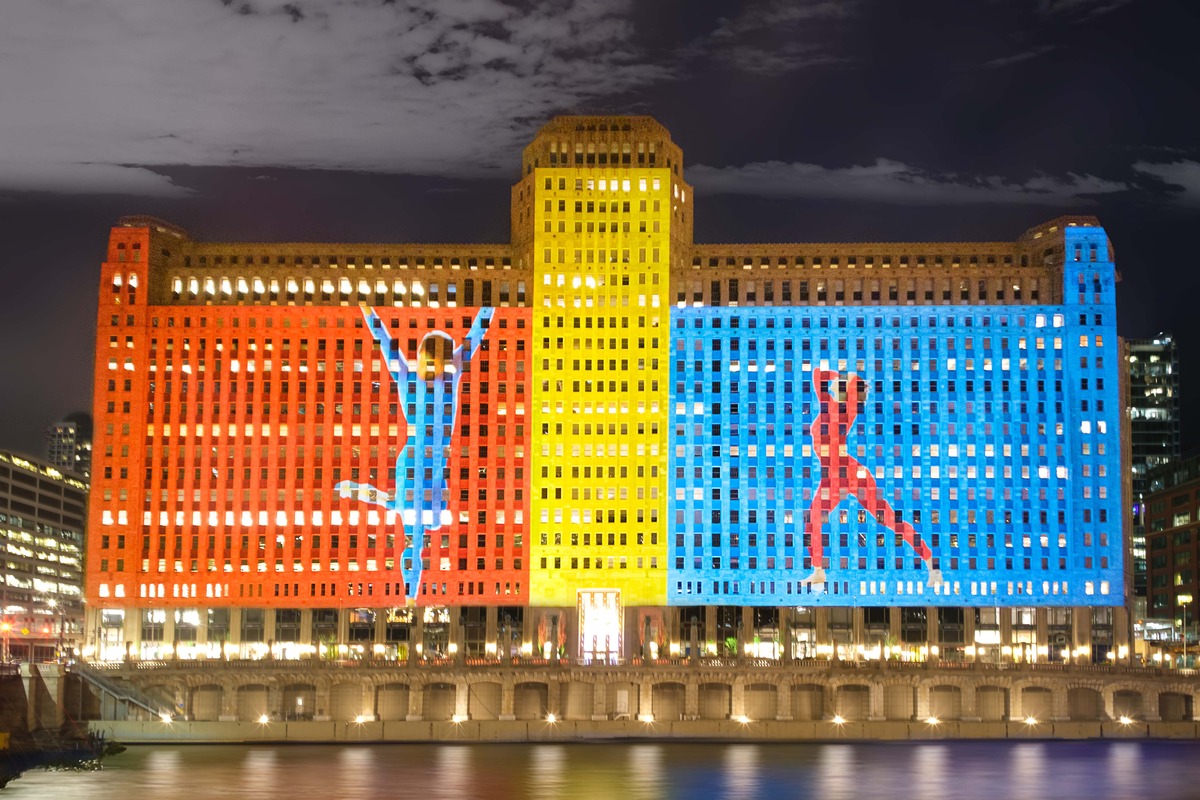This detailed photograph captures a prominent, approximately 20-story building at night, likely located in Paris and advertising the upcoming Olympics. The building, which could be a hotel, is brightly illuminated and features vivid, artistic murals of figure skaters on either side. The left side of the building is predominantly orange, showcasing a blue-clad male figure skater with his arms raised and leg bent behind him. The right side is painted a sky blue, depicting a red-dressed female figure skater in an elegant pose with both hands on her head and her body leaning to the left. Centrally, the building's yellow tower rises about five stories taller than the rest of the structure. In the foreground, a river and a walkway with arches and approximately 20-30 tan and brown pillars can be seen, adding to the picturesque scene. The backdrop features a black night sky with a few other buildings, lit up and ranging from five to 20 stories tall. Lights from the walkway shine upon the building, emphasizing its symmetrical, rectangular form and the striking Olympic-themed murals.